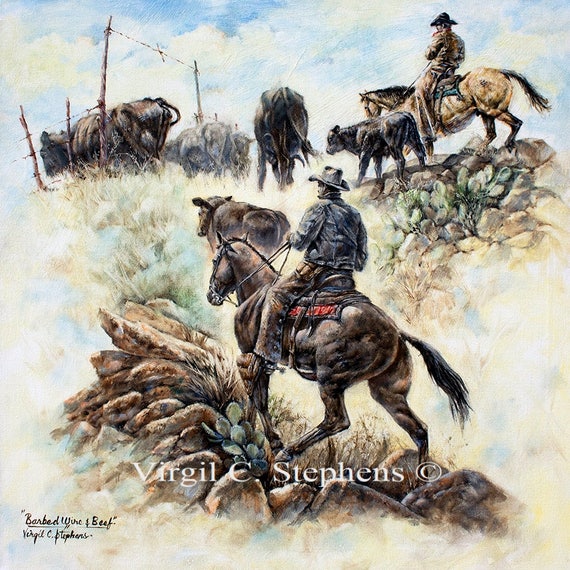The painting, titled "Barbed Wire and Beef" by Virgil C. Stevens, depicts a classic western scene rendered in a watercolor or possibly oil painting style. In the composition, two men, dressed in traditional cowboy attire with cowboy hats and jackets, are seen from the back as they ride their horses uphill. The cowboys are guiding a herd of cattle, consisting of bulls, cows, and a baby calf, towards a barbed wire fence. The cowboy in the foreground is donning a black hat and shirt with brown pants, while the other cowboy, positioned higher up the slope on a brown horse, is dressed in brown. The landscape features rugged terrain with rocks, cacti, grass, and wheat, set against a light sky with clouds. The foreground, where the men and animals are, is dark and defined, contrasting with the lighter, less detailed background. The painting is signed by the artist and bears his copyright watermark, emphasizing the authenticity of the artwork.